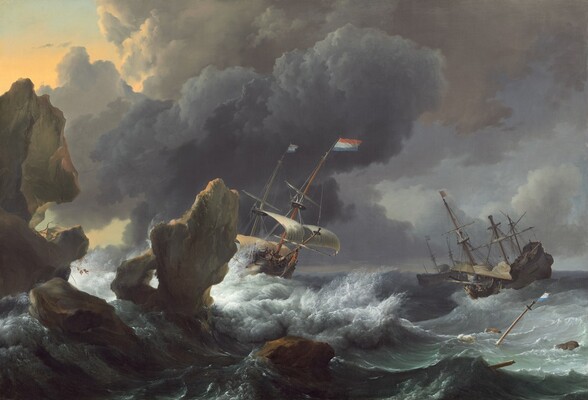A tumultuous ocean scene is vividly depicted in this side-angle painting, capturing the raw power of nature. The ocean is a churning mass of light-gray waves crashing high, their frothy crests mostly white with hints of gray. Against this backdrop, the dark gray clouds dominate the skyline, reaching down to about two-thirds of the painting. Patches of white clouds intersperse within, while a hint of blue and orange in the top-left corner suggests the beginning or end of the day.

In the foreground, jagged light-brown rock formations protrude from the ocean, their rugged surfaces weathered by the relentless waves. On the right, partially submerged and battling the stormy sea, is a gray ship with all its sails down, three masts standing prominent. It appears small and distant, adding a sense of scale to the vast, turbulent waters.

Midway into the painting, another ship angles towards the viewer, its front sail caught slightly sideways. This vessel features two visible masts, the foremost adorned with a tricolor flag of red, white, and green. Amidst the chaotic waves, nearly hidden, are the remains of another mast poking out from the water, possibly signifying a shipwreck.

To the left of this central scene, additional brown rocks extend off the page, amplifying the perilous environment. The drama of the painting is heightened by the suggestion of at least three ships fighting the storm, with one ship seemingly on a crash course with the formidable rocks, while another appears to be already succumbing to the sea's might.